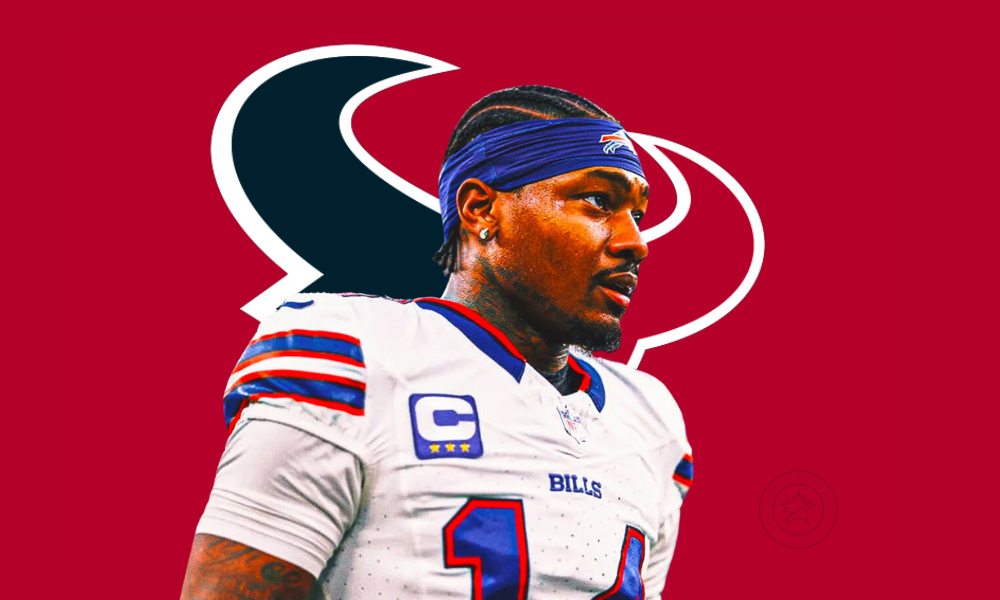In this detailed image, football player Stephon Diggs is prominently featured in his white Buffalo Bills uniform, accented with blue and red stripes on the shoulders. He is adorned with a blue headband that bears a symbol, and he sports a white diamond stud earring in his left ear. Diggs, a black athlete, has a short hairstyle with distinct lines between the hair, a small black mustache, and minimal chin hair, complemented by a noticeable neck tattoo. As a team captain, his jersey proudly displays a "C" with three stars below it in a blue box. The number "14" is visible on his jersey, along with the team name "Bills" across the center. His left arm has visible tattoos, while details on the other arm are indistinct. Behind Diggs, the background is predominantly red, featuring the blue and red Houston Texans logo at the center, adding contrast to the scene.